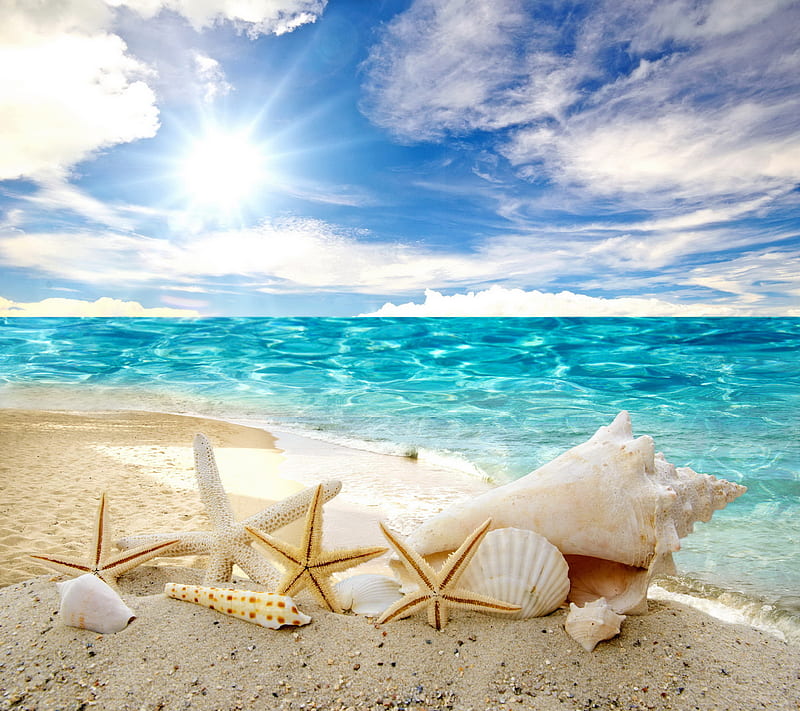The image depicts a serene beach scene with a detailed and varied foreground, including several crustaceans, shells, and starfish scattered across the sandy shore. Notably, the sandy area contains a mix of white and beige shells, one distinguished by brown square-like spots. A large conch shell is prominently positioned on the right, its tip facing the water, accompanied by three smaller conchs. In addition, there are starfish, including a yellow one with brown interior details and a bland white one.

The sand is textured with light and dark pebble-like grains, providing a natural, yet visually interesting base that extends towards the shore in the background. The water, which appears almost artificially vivid with shades of blue, enhances the ethereal feel of the scene, contrasting with the realistic beach elements. The background showcases the meeting point of water and sky, where the horizon draws the eye to a blend of blue skies and wispy, white clouds. The upper left corner is illuminated by a bright sun, completing the image with a warm, sunny atmosphere that feels both natural and slightly surreal.